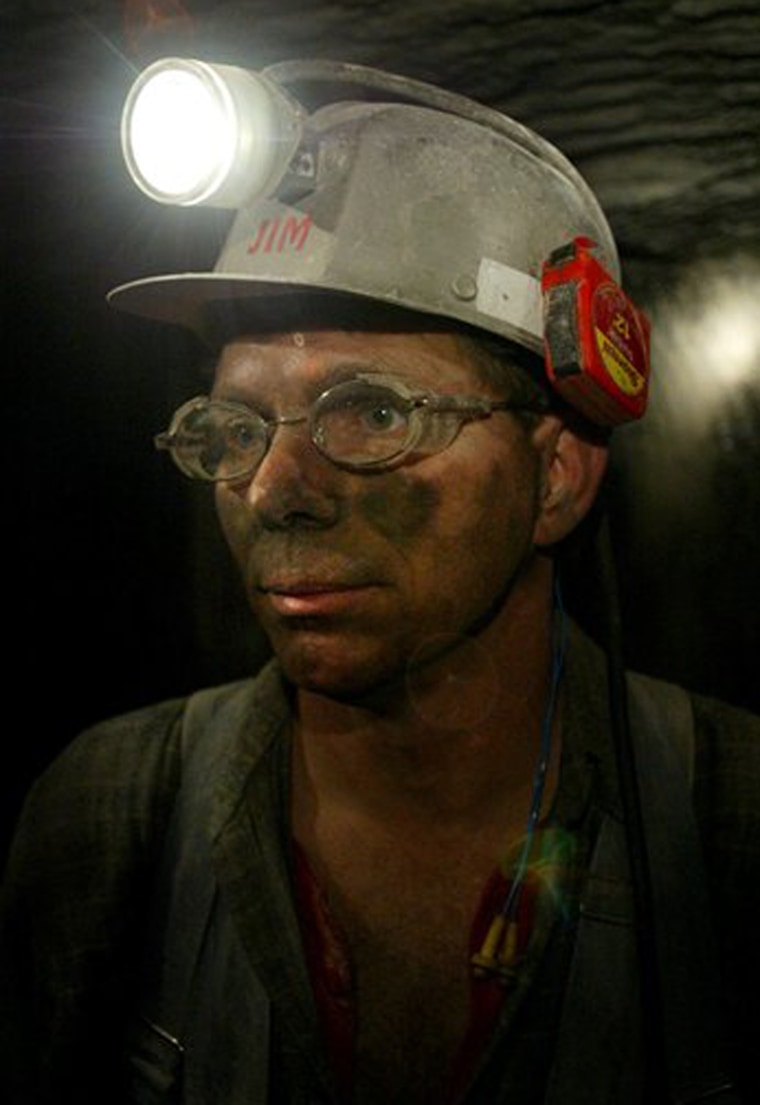In this image, a coal miner is depicted from the chest up, positioned centrally against a dark, cave-like background. The miner is wearing a hard hat with a bright white headlamp attached front and center, illuminating his face, which is smudged with dirt and grime. On the left side of his hard hat, a tape measure is secured, adding a touch of specificity to his gear. The miner’s eyes are protected by clear, industrial-style goggles that cover his glasses. He is dressed in dark clothing, including a partially unbuttoned shirt with visible shoulder straps. The ambient light from the headlamp highlights the miner's rugged features and work-worn attire, emphasizing the gritty, subterranean environment. The text "Jim" is displayed, possibly as a name tag or identifier. The color palette includes shades of beige, tan, red, black, gray, and a faintly noticeable greenish fuchsia, contributing to the realistic and somewhat somber tone of the scene.